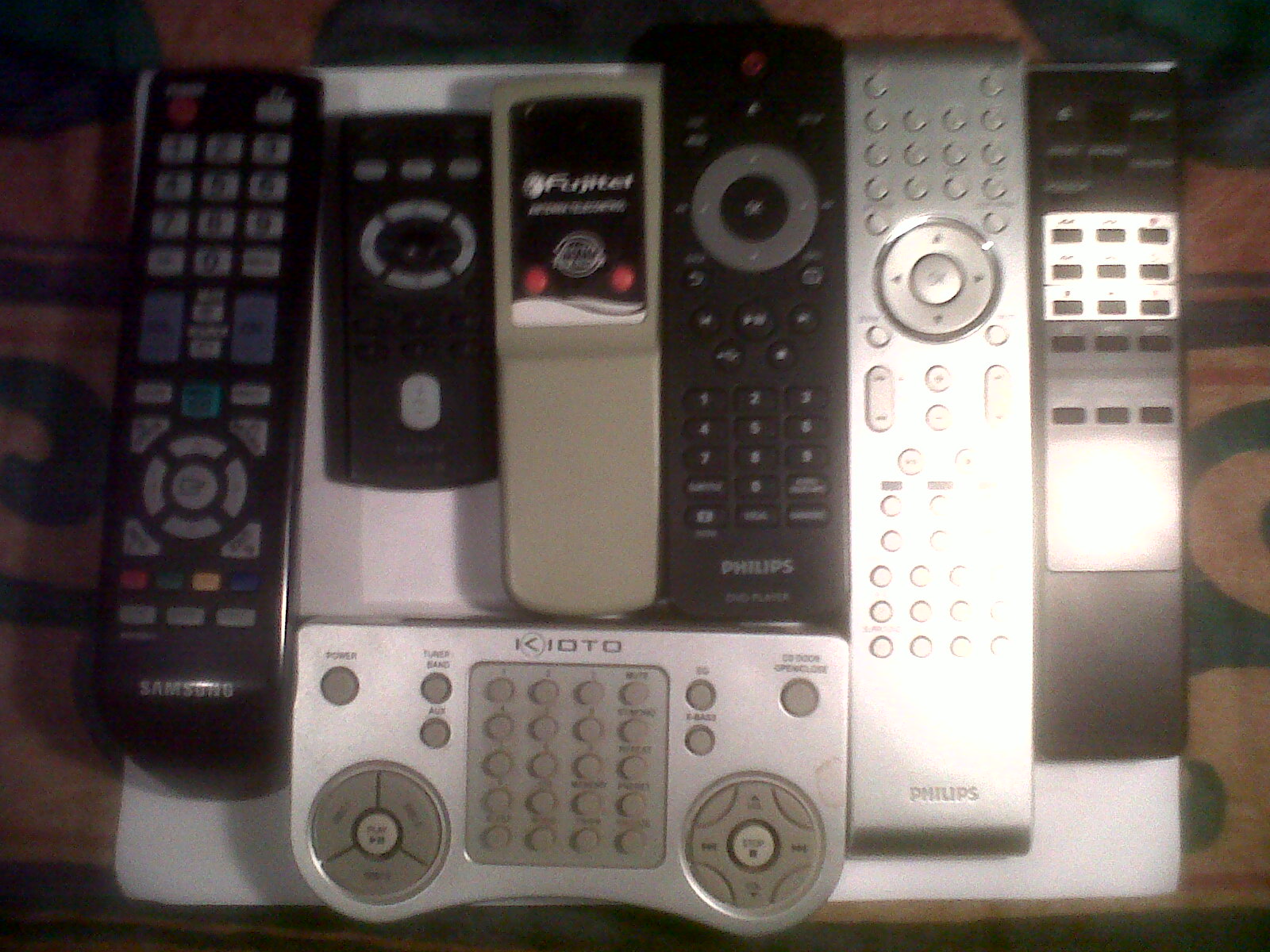This photograph showcases a collection of various-aged remote controls, predominantly from the 1990s to early 2000s, laid out on a light brown rug patterned with black rounded circles. The overall image is slightly out of focus with dark lighting, resulting in subpar image quality. On the left, there's a long black Samsung remote with predominantly gray buttons and a few red, yellow, and blue buttons, followed by another black remote featuring a circular button layout at its center. Next, a light gray remote with indistinct branding has two red buttons and a central gray logo. A black Philips remote with a red button at the top and a similar circular button pattern is placed beside another long, silver Philips remote. Adjacent to this, there is a black and silver remote with black buttons. At the bottom of the arrangement sits a Kyoto remote, characterized by its silver color and two prominent circular buttons on each side, along with an array of smaller buttons organized in a square formation. These remotes appear to be placed directly on the rug, which contradicts an initial observation suggesting they were on a white piece of paper on a table. Additionally, the supposed brown desk and remote holder seen by one viewer are not evident upon closer inspection.